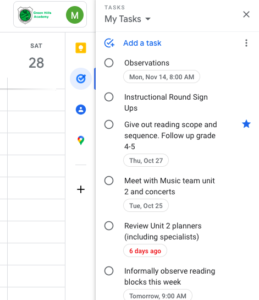This image displays a detailed task planner page listing various tasks and dates. At the top, it categorizes tasks and individual assignments alongside important dates, such as Saturday, October 28th. Notable entries include an 'Add a Task' section, observations scheduled for Monday, November 14th at 8 AM, and specific instructional activities like 'Instructional Round Sign-Ups', 'Distribute Reading Scope and Sequence', and 'Follow Up with Grade 4-5'. Additional meetings are noted with the music team to discuss units, performances, and concerts. An informal observation of written blogs is planned for tomorrow at 9 AM. The planner uses green, black, and yellow colors against a white background to highlight and organize information.